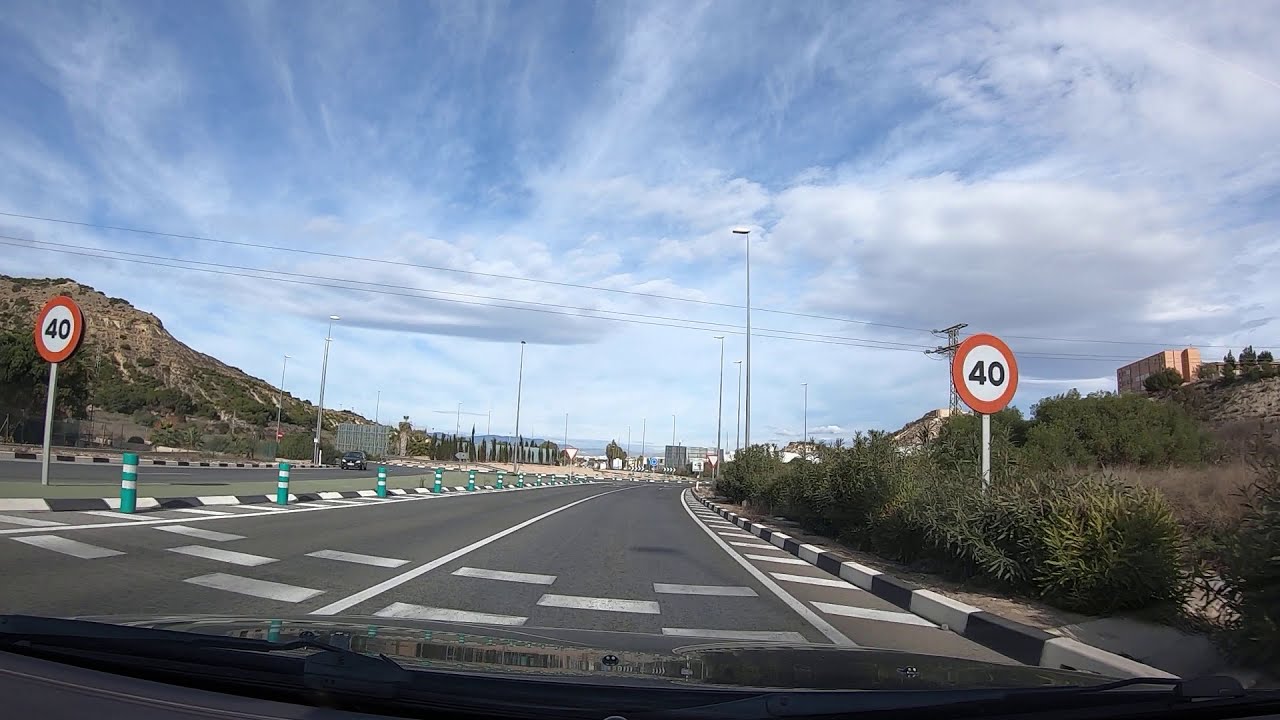The image captures a street view from inside a car, with the vehicle's black hood and dark gray dashboard framing the scene. The road ahead features a prominent white checkered crosswalk. Flanking the road are two white poles, each displaying a round, white sign bordered in red with the number "40" in black. To the left, there are green pillars with white stripes lining the street, alongside a large hill dotted with green trees and shrubbery. The right side showcases green vegetation, several bushes, and a square rectangular building further back. The road edges are marked by a black and white striped curb. The sky above is a bright, light blue adorned with a mixture of wispy and thick white clouds, suggesting a clear and sunny day. No other vehicles are visible in the distance, adding to the tranquil scene.